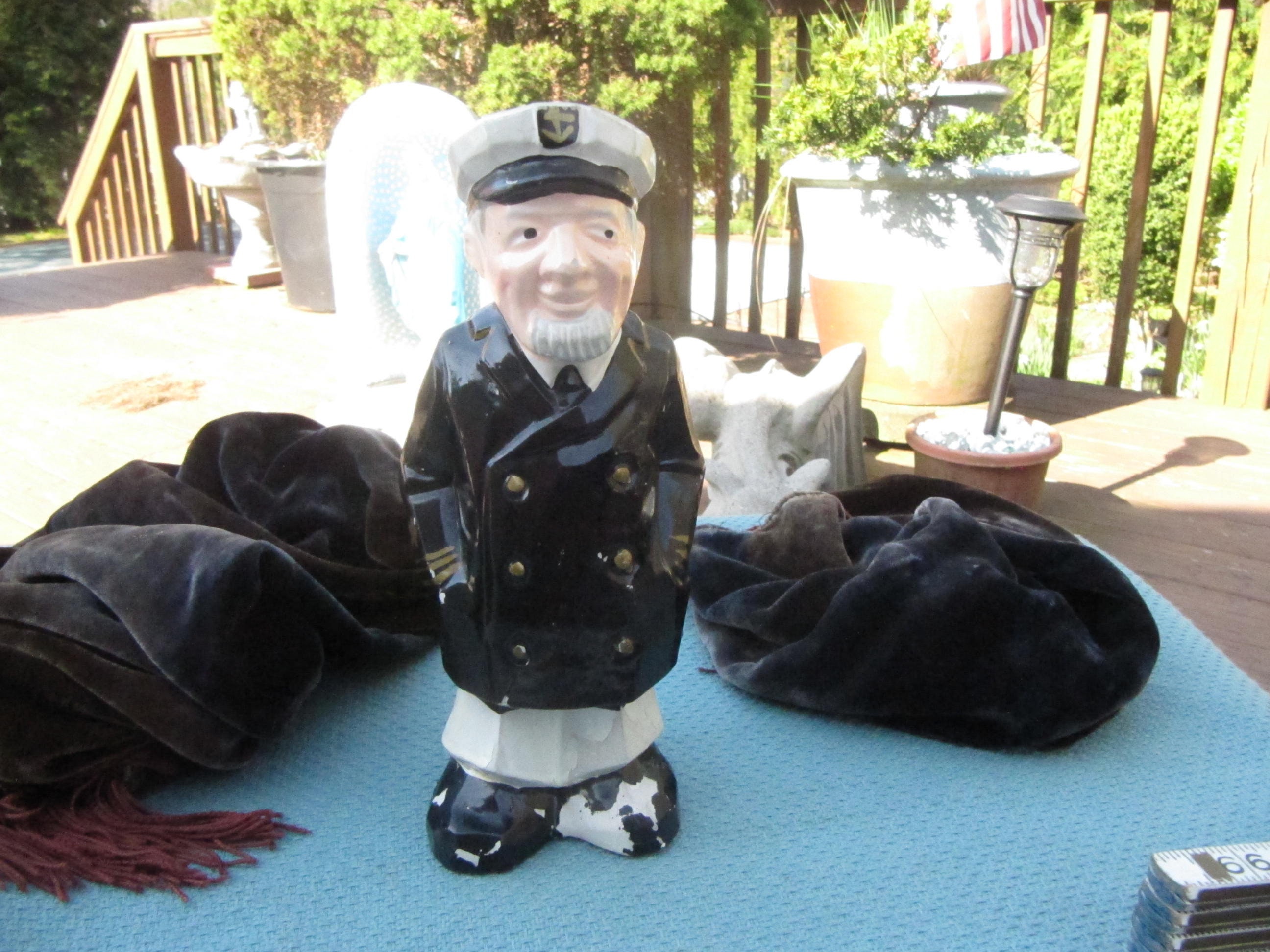In this detailed, photographic image set outdoors, we see a weathered ceramic figurine of an older sea captain. The figurine, displaying a cracked, chipped surface, especially noticeable on its feet, is adorned in a dark peacoat with gold buttons, white pants, and black shoes. The captain wears a pristine white hat, marked with a black rim and possibly an anchor emblem, and sports a white beard. His hands are tucked into his coat pockets as he gazes slightly upward with a subtle grin.

The scene is set on a hardwood porch, adorned with various elements. Surrounding the captain are two black blankets, one with tassels, lying to his left and right. Behind him, a large planter houses a solar lantern. Another planter, described as coral-colored, also contains a light. Further back, there is a wooden porch railing and a stairway leading downwards, with green plants basking in the sunlight beyond. The end of a ruler, marked with the number 66, can be seen at the bottom right of the image, the only textual element present in the photo.

The entire setup rests on a textured, light-blue blanket that covers part of the wooden surface of the porch. The background is filled with green foliage, providing a lush, natural backdrop to this intriguing and evocative scene.